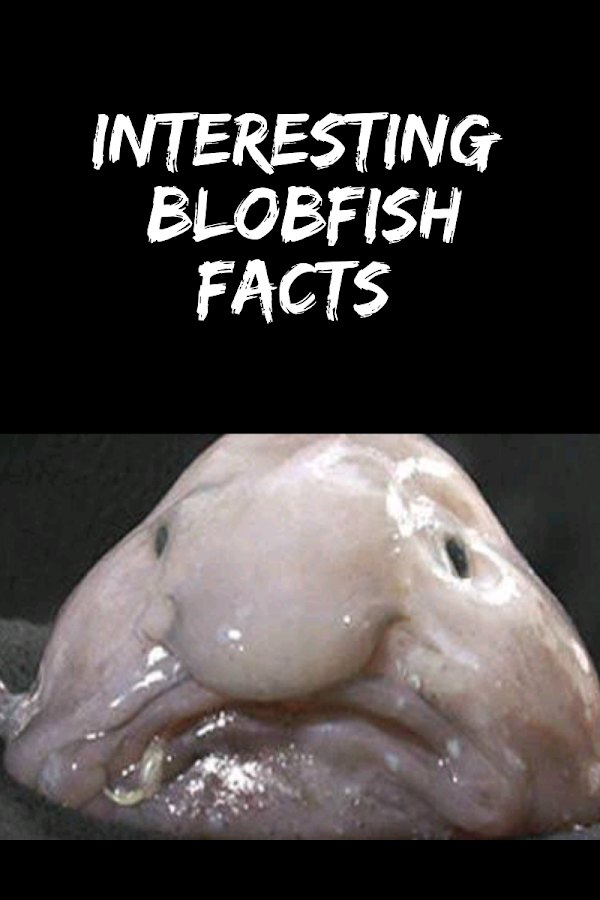The image is divided into two sections. The top half features a solid black background with white, all-caps text that reads "INTERESTING BLOBFISH FACTS" in a brushed-like font. Below this text, the second half of the image showcases a picture of the blobfish, a notably unattractive creature. The blobfish has a beige to pinkish, somewhat translucent, and slimy appearance with a face resembling that of a very sad or frowning old man. Its face, which is roughly shaped like a rounded triangle, prominently features two small, elongated black eyes situated on either side of a large, blob-like nose. The creature's mouth also adds to its mournful expression, appearing almost human-like in its contours.